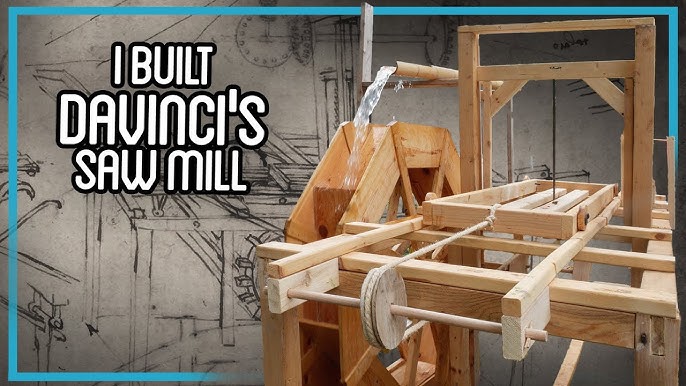The image appears to be a YouTube thumbnail showcasing a meticulously constructed wooden sawmill inspired by Leonardo da Vinci's designs. The background features gray and white blueprint-style sketches that provide a detailed outline of the contraption. Boldly displayed across these blueprints, in a unique white font with a black border, is the title: "I built Da Vinci's Sawmill." Dominating the right side of the image is the wooden sawmill itself, which includes various intricately assembled components such as pulleys and ropes. A prominent feature is the water wheel, fed by a half-open tube at the top, where water flows through to drive the mechanism. A long, thin black line, likely a saw blade, is vertically supported by the wooden frame, hinting at the operational part of the machine. The sawmill, constructed from both lightly and darker shaded wood, stands as a tangible realization of the detailed schematics in the background, effectively merging historical design with modern craftsmanship.